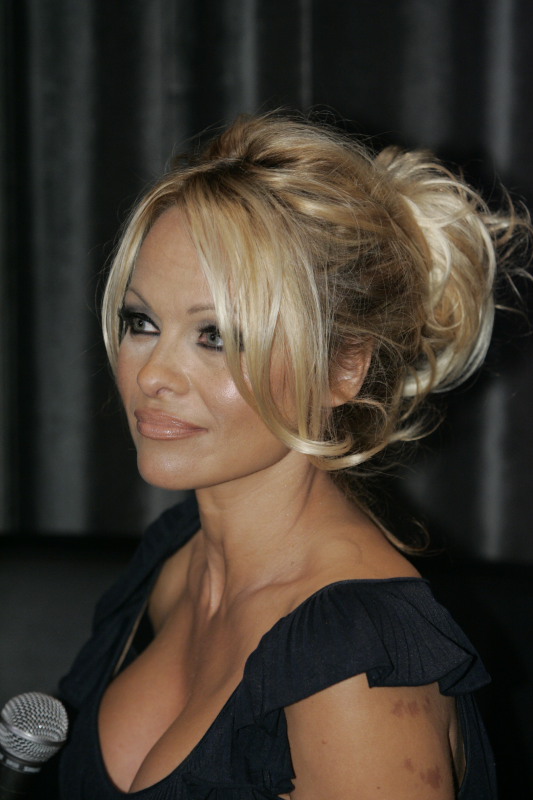In this image, the primary focus is on Pamela Anderson, who appears to be in her 40s. She is standing in the center of the frame, facing sideways towards the left. Pamela has long, dirty blonde hair styled into a large messy bun at the back. Her complexion is very tan, and she is wearing black eyeliner, eye shadow, and light pink lipstick. Her attire consists of a black top with short sleeves, revealing some cleavage.

Behind her is a backdrop of black curtains, adding a dramatic contrast to the scene. In the bottom left corner of the image, the silver head of a microphone can be seen, suggesting that she might be preparing to give a speech or address an audience. The setting is not explicitly described but implies a formal or semi-formal occasion. Notably, Pamela has some bruising or scar tissue on her arm, adding a touch of realism to this poised image.